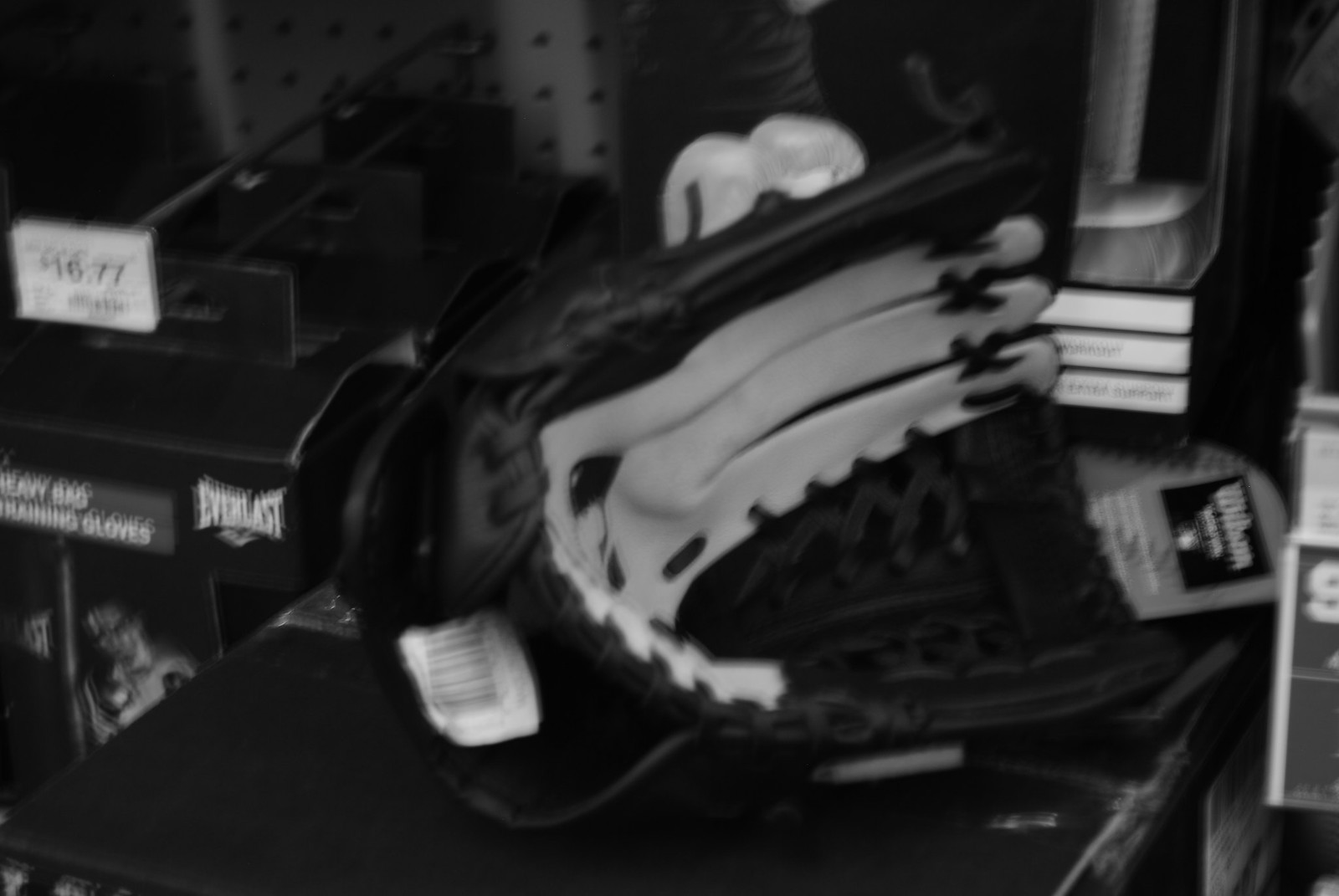This out-of-focus black and white image, taken in what appears to be a Walmart or a sporting goods store, features a display setup with pegboard hooks visible due to the evenly spaced holes on the wall. Prominently displayed is a dark-colored leather catcher's mitt, likely a Wilson based on a partially visible insignia on the right. To the left, a metal display hook supports a mostly white price tag marked $16.77, indicating the cost of nearby Everlast gloves, packaged in dark cardboard containers. There's a faint image of a baseball player wielding a bat on one of the boxes, enhancing the sporting theme of the scene.